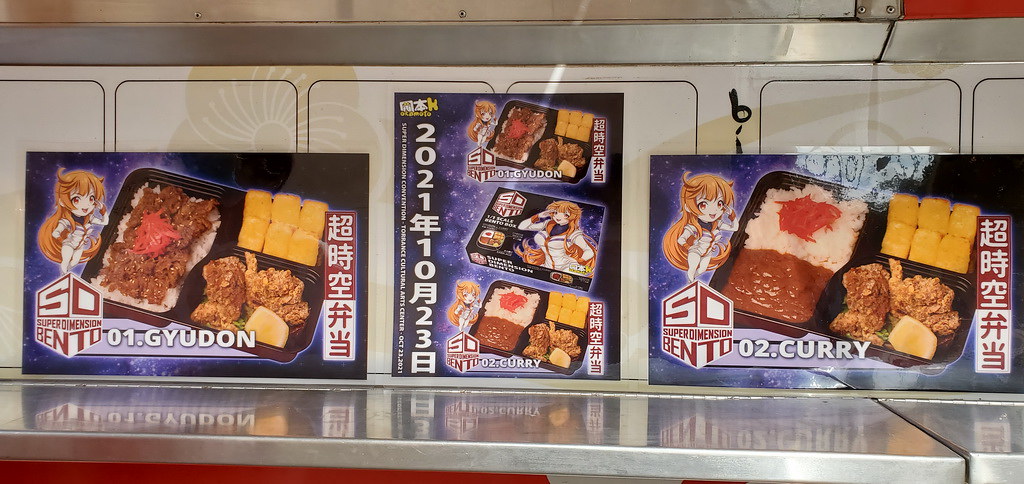This indoor photograph captures a section of a restaurant featuring three rectangular posters attached to a glossy, reflective steel countertop and a metallic wall. The metallic wall is white and grey in color, and the posters are advertisements displaying various food items. Each poster follows a similar design theme with slight variations.

The leftmost poster has a black and purple background and features a food plate placed in the center, accompanied by an anime character to its left. Below the image, it reads "SD Super Dimension Bento 0.1 Gyudon," with additional text written in Japanese. The middle poster shows three food plates—one covered and two open— with the same anime character present and Japanese text. The rightmost poster mirrors the design of the left poster but instead reads "02. Curry."

Collectively, all three posters highlight different menu items with detailed visuals and text in Japanese, complemented by the consistent image of an anime girl with orangish hair, and are designed to attract attention with their vibrant colors and clear illustrations.